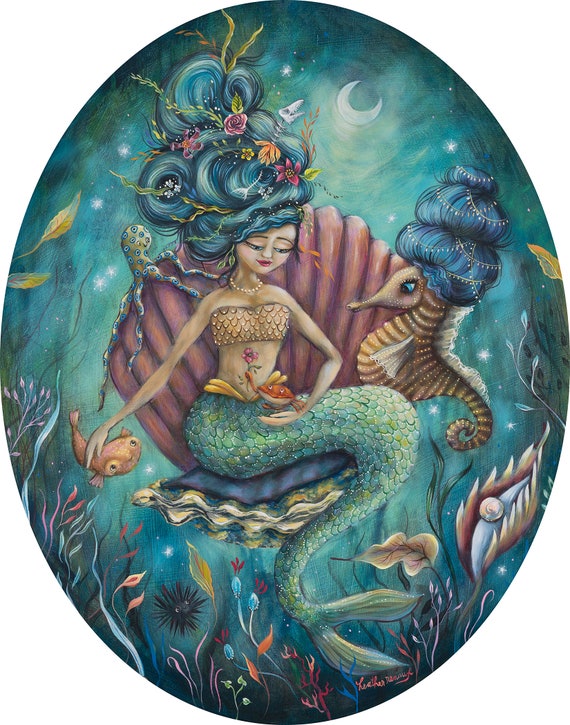The image is an oval-shaped painting of a mermaid, set against a vibrant oceanic background with varying shades of blue. The mermaid sits gracefully atop an open clamshell that transitions from pink to orange hues. Her bottom half features vivid lime and peacock green scales, forming a sleek fish tail, while her top half is covered with a tan crop top made of similarly shaped scales. Her abundant blue hair is styled into an elaborate bun adorned with fish bones, flowers, seaweed, and kelp.

One of her hands delicately holds a small orange crab that presents a pink four-petal flower, while the other hand strokes a deflated pufferfish on her lap. A large, tan, and brown seahorse with golden hints and three tiers of striking purple-blue hair, decorated with fine ropy jewelry, floats to her right. Surrounding the mermaid are various aquatic plants, wavy green grass, and additional sea creatures including a yellow octopus with blue rings and a hidden sea urchin.

Above the scene, a crescent moon, embellished with flowers in its hair, glows softly. The corners of the painting fade into a featureless white, drawing focus to the enchanting underwater tableau.